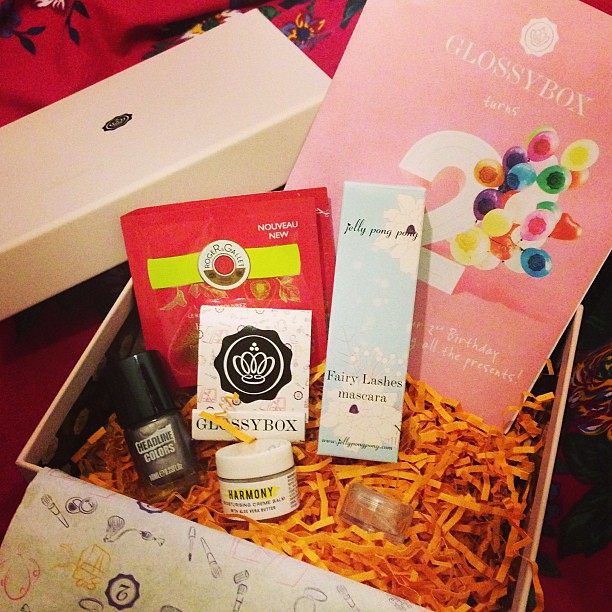The image shows an intricately arranged Glossy Box gift set, designed as a birthday present. The open box reveals a vibrant assortment of cosmetic items nestled in orange crinkle paper, resembling festive confetti. At the forefront, a floral-embellished face mask bearing "21" sits prominently, hinting at a celebratory 21st birthday. Next to it, a card further indicates the birthday theme. The items include a mascara, a lipstick or lip gloss box, a container of headline colors, bags of tea, nail polish, and a small travel-sized scrub. The lid of the box, adorned with the Glossy Box logo, rests against the upper left corner of the image. The box itself and the products, labeled with the brand name Glossy Box, suggest this scene is part of an advertisement for the brand's specialized birthday gift packages. The box is placed on a red tablecloth with a floral pattern, enhancing the festive atmosphere.